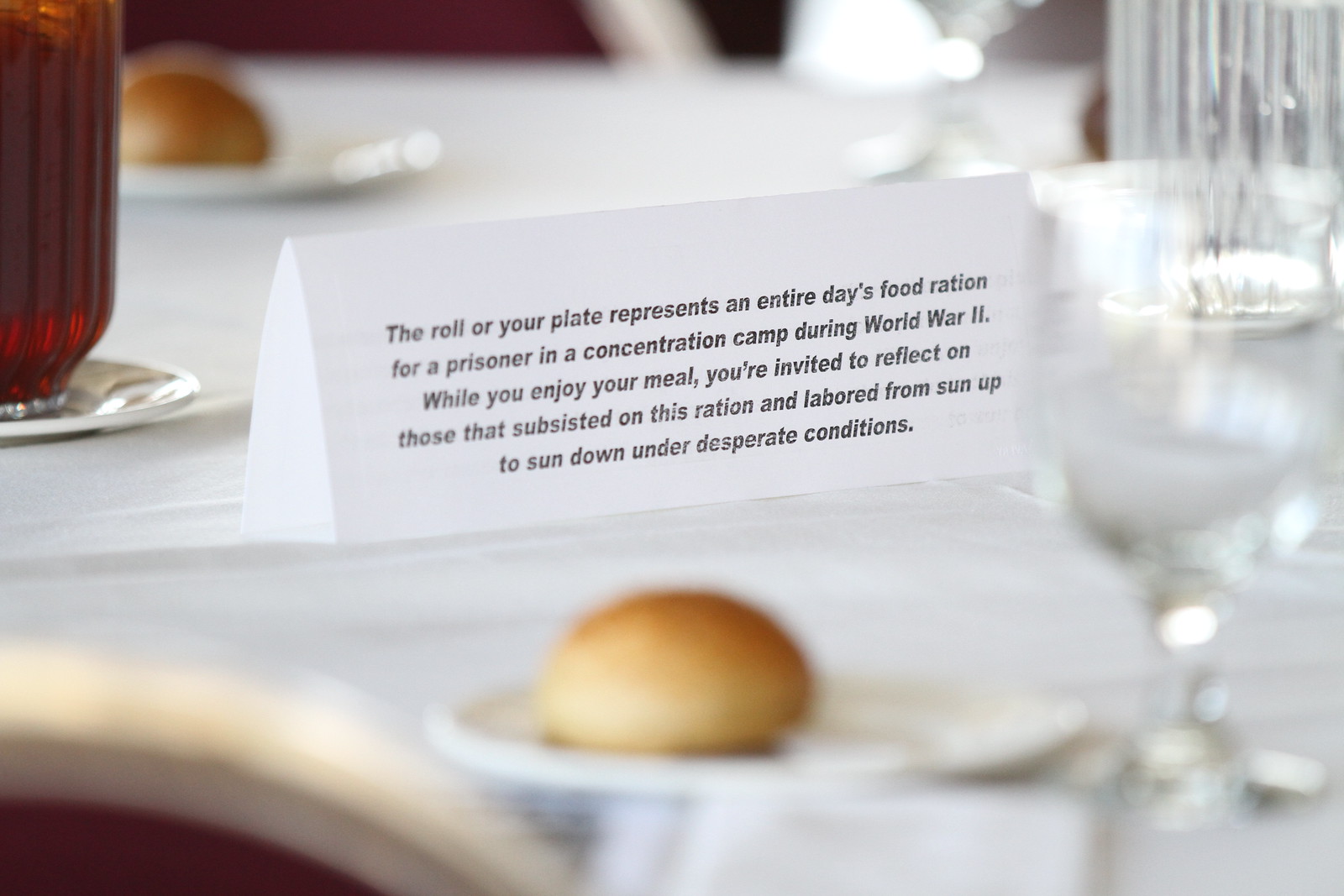The photograph captures an indoor setting, likely a restaurant, featuring a dinner table adorned with a white tablecloth and a variety of meticulously arranged items. Positioned across the table are empty crystal wine glasses and several small plates, each bearing a standard round dinner roll. A few dishes can be seen, including one that's slightly blurry in the bottom left, possibly a bowl. Dominating the center of the photograph is a conspicuous white folded piece of paper standing upright, upon which an important message is inscribed: "The roll on your plate represents an entire day's food ration for a prisoner in a concentration camp during World War II. While you enjoy your meal, you are invited to reflect on those that subsisted on this ration and labored from sunup to sundown under desperate conditions." The photograph's focus is clearly on this note, leaving most of the table slightly out of focus. The prominent colors in the image are black, white, red, and tan, contributing to a clean yet somber atmosphere that underscores the poignant reminder conveyed by the note.